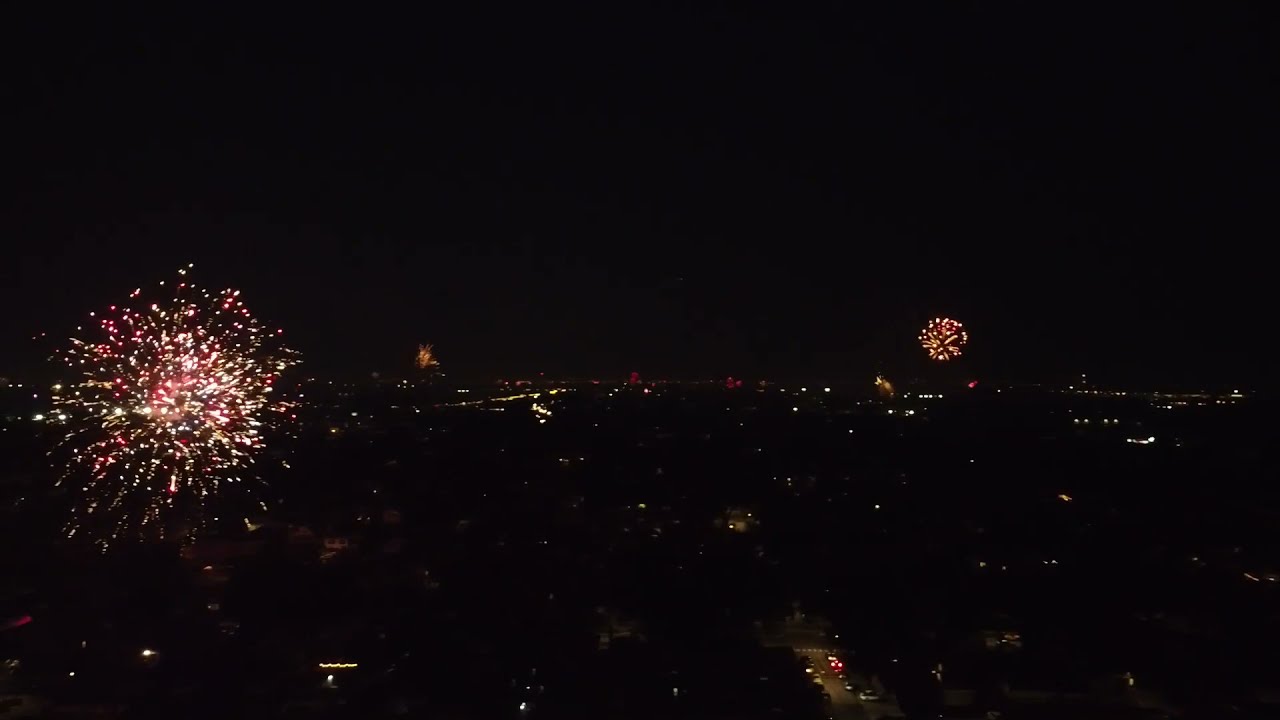This striking nighttime photograph, likely taken from a drone at a very high angle, captures a panoramic view of a city illuminated exclusively by its myriad lights and festive fireworks displays. The expansive black sky dominates the upper half of the image, devoid of stars, focusing all attention on the brilliant fireworks. In the lower portion, the glowing lights from buildings and roads form a soft, yellow-tinged web, threading through what appears to be a densely tree-covered area. Scattered throughout the dark expanse, multiple fireworks burst in an array of red, green, yellow, and white, suggesting a major celebration such as New Year's Eve or the 4th of July. The largest firework dazzles on the left side of the image, while smaller bursts pepper the horizon, adding depth and a sense of simultaneous revelry throughout the city. The dynamic contrasts between the vivid, colorful explosions and the serene, dimly lit urban landscape below create a captivating scene of celebration and beauty.